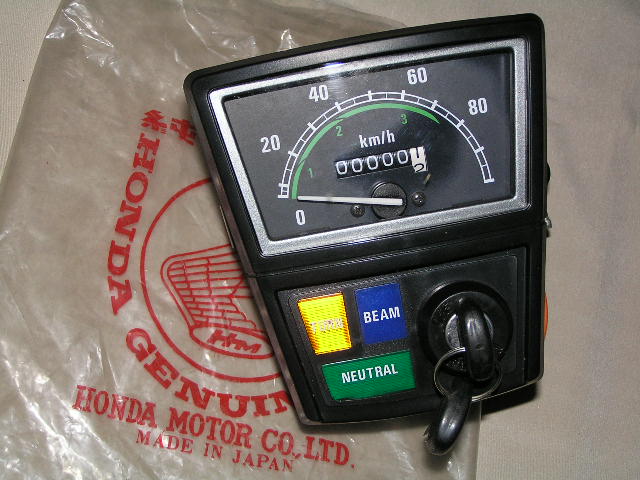This photograph features a close-up view of a rectangular, black device placed on a surface, which appears to be a tabletop covered with a plastic bag. The plastic bag is adorned with the Honda Gold Wing logo in red and includes the text "Honda Genuine" and "Honda Motor Co., Ltd., made in Japan," although some parts of the text are obscured.

The focal point of the device is a large meter situated on its top half. The meter is labeled "KM/H" and is scaled in increments of 20, 40, 60, and 80, with the scale ranging from 0 to 100, though the 100 mark is unlabeled. It features a white pointer currently positioned at 0. The meter also includes an odometer, which shows a reading between 1 and 2. 

The meter's curved scale is mostly white with gradations at every 10 KPH and smaller markers at every 5 KPH. There is a green section on the scale marked with values 1, 2, and 3 beneath the main graduation, extending up to around 70 or 75 KPH.

At the bottom of the device, there is a visible key inserted into it. Adjacent to the key are buttons labeled "Beam" in blue and "Neutral" in green, alongside a yellow light indicator.

The composition and the details of the photograph suggest that this device might be part of the instrumentation or control system of a Honda Gold Wing motorcycle.